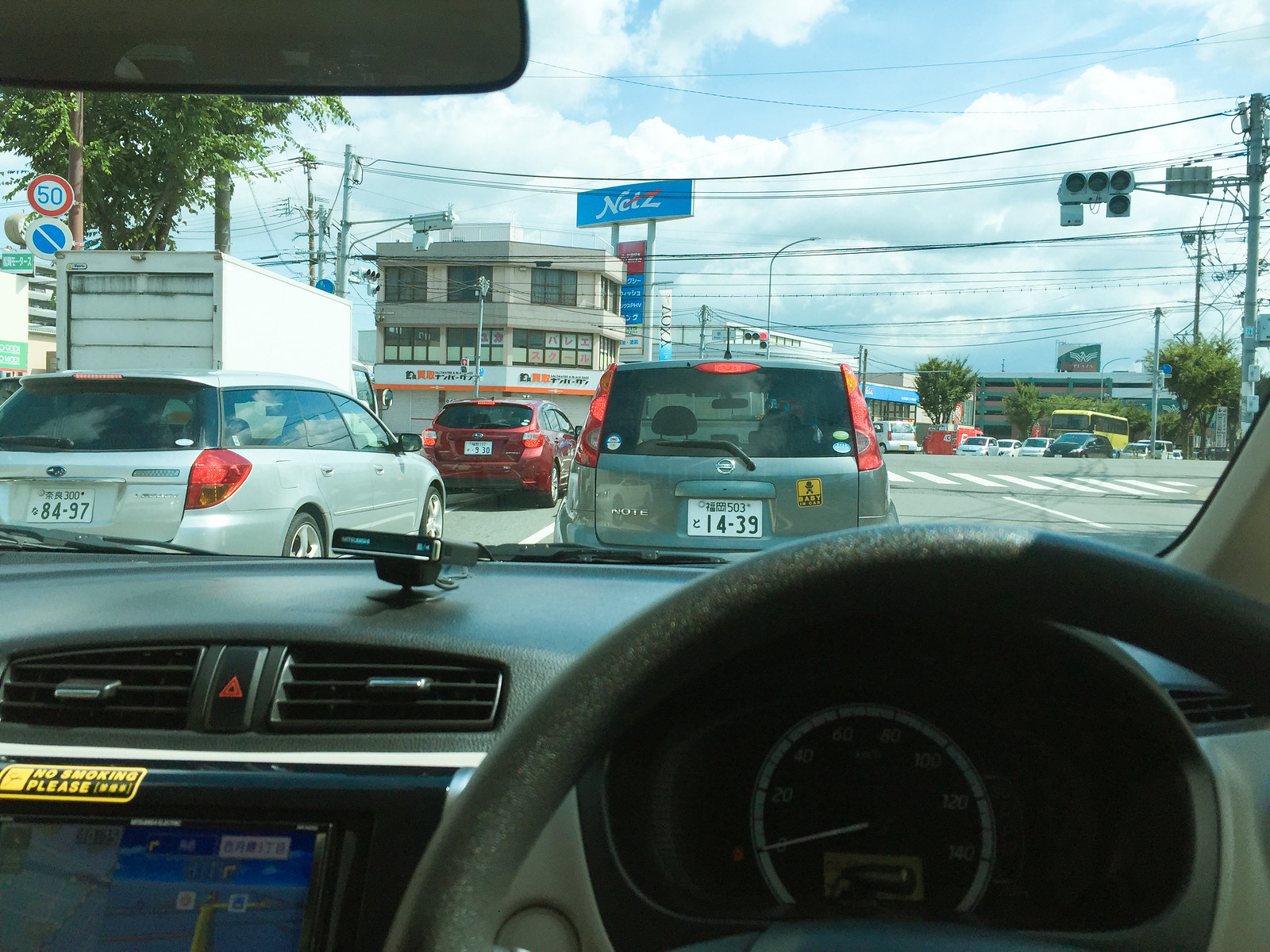The image, taken from inside a right-hand drive car, captures a busy intersection scene filled with details. The vehicle is surrounded by a diverse array of other automobiles, including a silver SUV directly ahead, a red car, a silver car, a large white box truck to the left, and a yellow bus. The car's rearview mirror is visible in the left corner of the image, along with a 'no smoking please' sticker, air vents, and a navigation system on the dashboard. The sky above is blue with numerous white clouds, and the street is populated with traffic lights, stop signs, power poles with lines strung overhead, and a variety of signs in a foreign language, indicating this is likely a country where driving is on the left side. Prominent features include a tannish brown building with orange signage above the red car and white license plates with black numbers on the vehicles. In the background, tall buildings form the skyline, adding to the urban landscape filled with bustling activity.